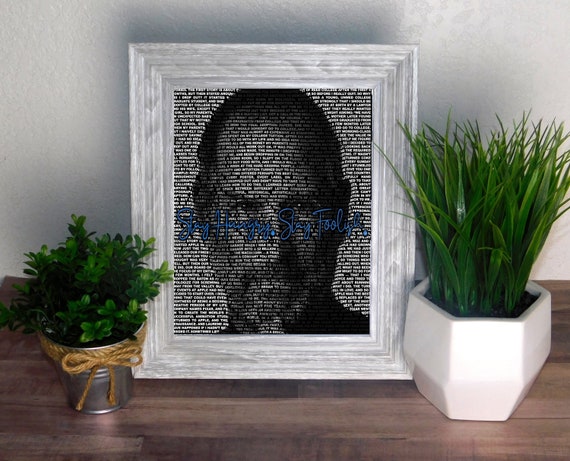In this framed photograph, an intense black and white image of Steve Jobs stares piercingly at the viewer. The photograph is unique, composed of numerous tiny, unreadable words, creating a pixelated texture. Bold blue cursive scrawls "stay hungry, stay foolish" across the center of Jobs' face, adding an inspirational touch. The picture is enclosed in a weathered white wooden frame, resting on a dark wood table, positioned against a gray wall, suggesting a home setting. Flanking the photograph are two small house plants—a taller plant with green shoots in an octagonal white vase on the right, and a shorter, bushier plant in a metal tin with a brown ribbon around the pot on the left—adding a touch of organic charm to the tableau. This setup seems to serve as a motivational reminder, encouraging not just perseverance but also a sense of balance and wisdom.